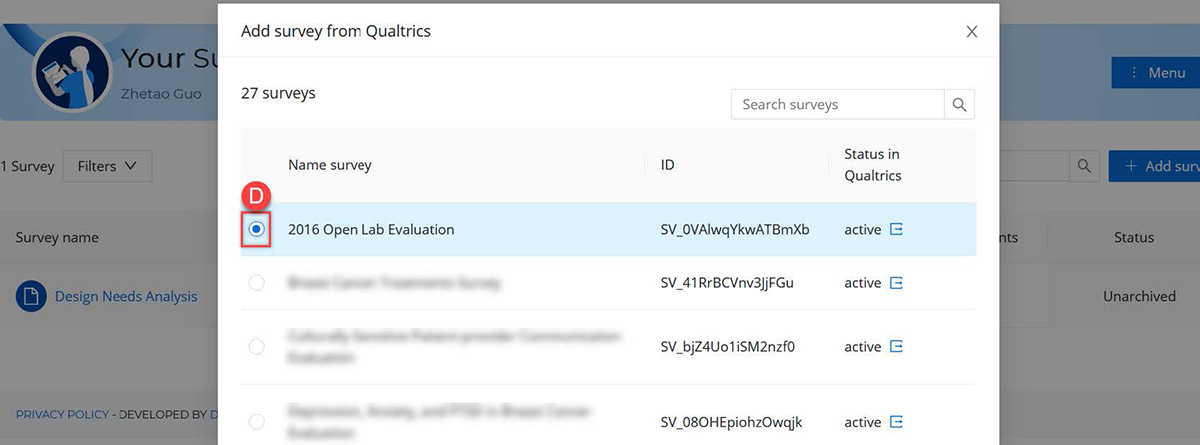The image is a screenshot of a website featuring a central pop-up window with a predominantly white background. At the top left corner of this pop-up, in bold black lettering, is the title "Add Survey from Qualtrics," with an elegantly styled capital 'Q' for Qualtrics. To the top right of the pop-up, a conspicuous 'X' suggests an option to close the window. Just below the title, the text "27 Surveys" is prominently displayed, with the numeral "27" for clarity.

On the right side beneath this, there's a search bar labeled "Search Surveys," accompanied by an icon of a magnifying glass. As you move down the pop-up, categories such as "Name," "Survey ID," and "Status" in Qualtrics are listed in a horizontal layout.

Directly below the "Name" heading, a blue banner spans the width of the pop-up. Encircling this banner is a red border, and there's a red circle above it containing a capital 'D' in white. Inside the blue banner, a smaller blue circle with a white border appears, hosting another blue circle within it. The text "2016 Open Lab Evaluation" is prominently featured here, while other survey names are blurred out for privacy.

In the background, partially obscured by the pop-up, the website’s interface displays a blue banner at the top. Within this banner is a small circular icon depicting a cartoon user avatar labeled with "UR," though this part is mostly hidden behind the pop-up window.